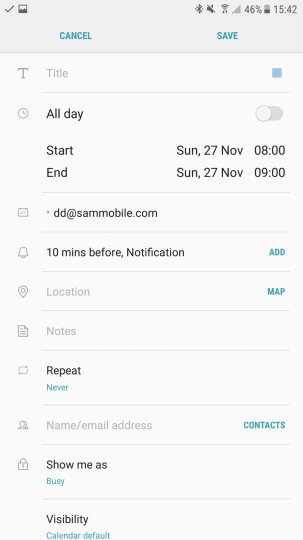The image is a detailed screenshot of a smartphone screen showing the setup for an alarm or a calendar event. At the top of the screen, several status icons are displayed: a check mark, a Bluetooth enabled icon, a mute volume icon, a battery usage indicator at 46%, signal bars for cell phone service, and the time, which reads 15:42. There is also blue text for the options "Cancel" and "Save."

The primary section of the screenshot reveals the interface for setting up an event or alarm. There is a field to add a title and a clock to set the duration of the event. The event is scheduled to start on Sunday, November 27th at 8:00 AM and end on the same day at 9:00 AM. Additionally, there is a bell icon for setting a notification 10 minutes prior to the event, an icon to add a location, an icon to add notes, and arrows indicating the option to repeat the event. You can also add a name or email address from your contacts. Lastly, a padlock icon is shown which, when clicked, reveals options for setting your status, with "Busy" selected by default.